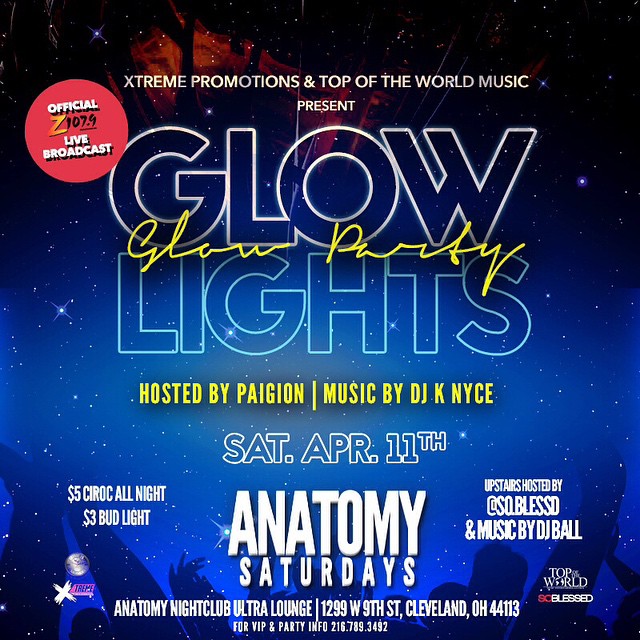This advertisement for the Anatomy Nightclub's "Glow Party" is vibrant and dynamic, beginning with a gradient background that transitions from a black night sky at the top to a deep blue hue filled with stars at the bottom. At the top in white text are the words, "Extreme Promotions and Top of the World Music Present." The central focal point features the phrase "Glow Lights" in a neon-style, outlined in white, with the words "Glow Party" elegantly written in yellow cursive nestled between "Glow" and "Lights."

In the upper left corner, a red circle prominently features the text "Official Z107.9 Live Broadcast," partially covering the "G" in "Glow." Just below the main title, information in yellow text indicates that the event is "Hosted by PAIGION" and "Music by DJ KNYCE." 

Further details about the event include the date, "Saturday, April 11th," which is displayed in a white outline font. Below this, "Anatomy Saturdays" is proclaimed in an elongated white font. The left side advertises special drink prices: "$5 Ciroc All Night" and "$3 Bud Light." On the right, it notes that the "Upstairs [is] hosted by So Blessed" with "Music by DJ Ball."

At the bottom of the advertisement, the footer provides the event location and additional contact information: "Anatomy Nightclub Ultra Lounge, 1299 West 9th Street, Cleveland, Ohio 44113," followed by a line for "For VIP and Party Info" with the phone number "216-719-2492."